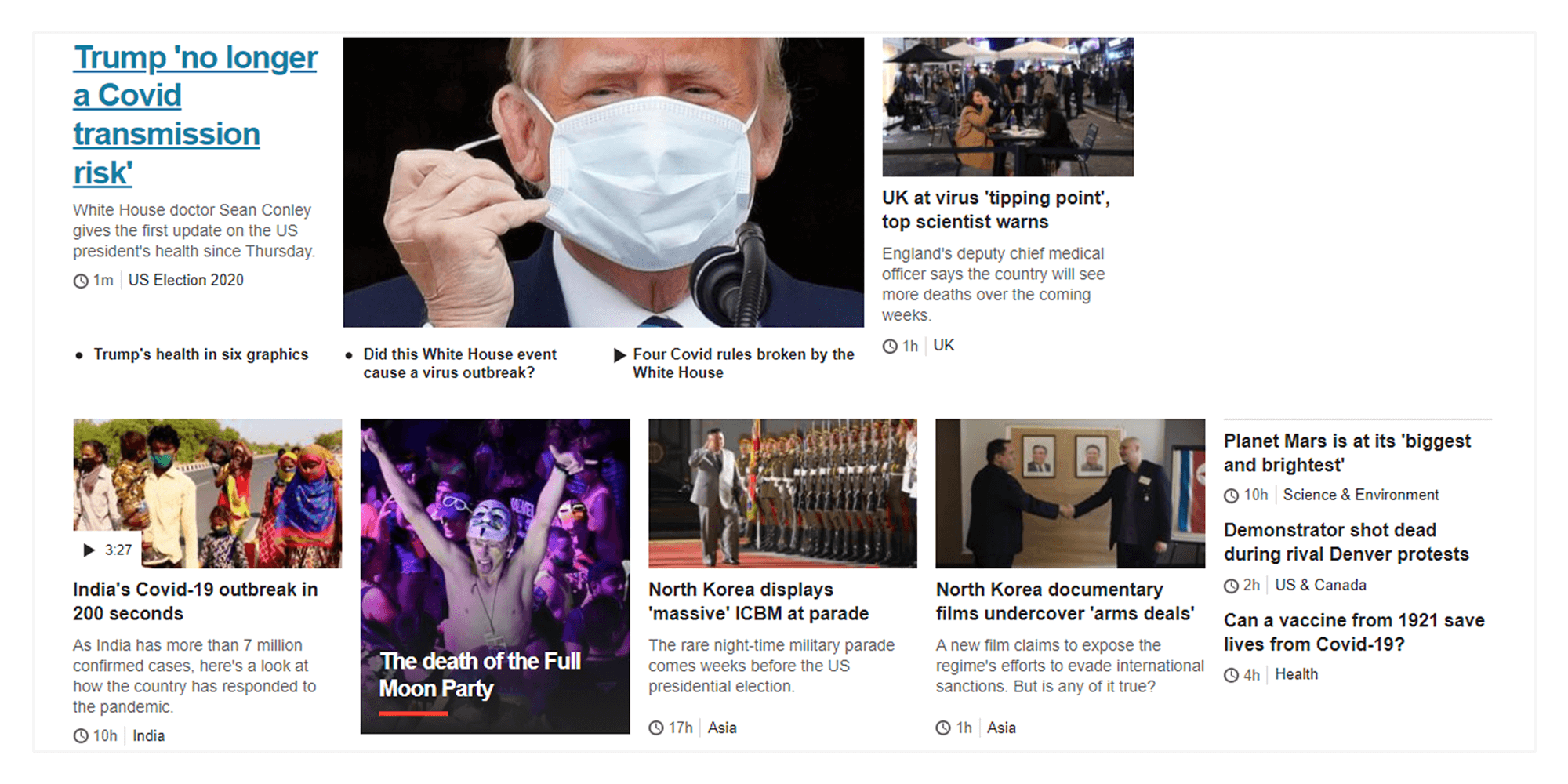This image is a screenshot of a news compilation displaying multiple articles arranged in two rows. 

The top row features three articles: 
1. "Trump No Longer a COVID Transmission Risk"
2. "Did This White House Event Cause a Virus Outbreak?"
3. "UK at Virus Tipping Point, Top Scientists Warn"

Each of these articles is accompanied by a title, a brief description, and the date they were last updated or loaded.

The bottom row contains four different images and an additional column listing three separate articles:
1. "Planet Mars is at its Biggest and Brightest"
2. "Demonstrators Shot Dead During Rival Denver Protests"
3. "Can a Vaccine from 1921 Save Lives from COVID-19?"

Overall, the screenshot captures a diverse array of news topics ranging from political and scientific developments to current global events.